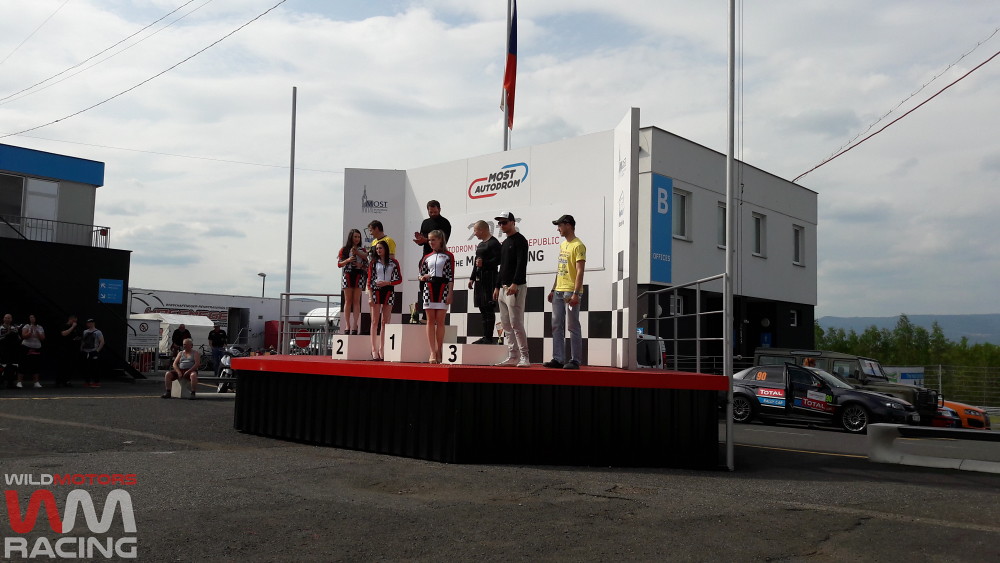The photograph captures an awards ceremony set on a raised stage with a red floor, featuring three podiums numbered 1, 2, and 3, with the center podium being the tallest. Standing proudly on the podiums are four individuals: two women in white vests adorned with black and white checkered patterns, and two men in white shirts paired with black hats. The stage is framed by a black curtain and accented with silver poles and drawstrings on either side. In the backdrop stands a two-story building, black on the bottom and white on the top, with an emblem reading "Most Autodrome" at the center, beneath which a flag hangs. The "Most Autodrome" logo is distinguishable by its blue and red semicircle. Overcast skies with white and gray clouds loom in the background, and a variety of race cars, including a black car covered in advertisements and a nearby jeep, line the right side of the building. In the bottom left corner of the image, the words "Wild Motors" are visible, with "Wild" in white, "Motors" in red, and a merged "W" and "M" symbol, the "W" in red and the "M" in white, below which "Racing" is printed in gray letters. This scene likely celebrates the conclusion of a racing event, recognizing the top competitors on the podium.